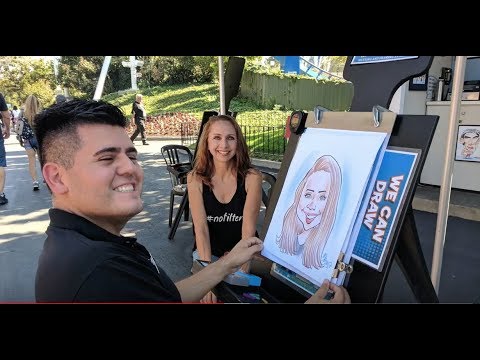In this vibrant outdoor photograph, a cheerful male artist, clean-shaven with neatly groomed short brown hair, and dressed in a black short-sleeved collared shirt, sits at his drawing board on a sunny day. He proudly displays his recently completed caricature of a smiling young woman with reddish-blonde hair, who sits across from him in a sleeveless black tank top emblazoned with the white text "no hashtag no filter." The caricature, drawn on a large white pad, humorously exaggerates her features in typical caricature style. Telling details suggest this image may be a screenshot from a video, framed by black bars at the top and bottom and intersected by a red line above the lower bar, resembling a progress bar from YouTube. The scene is lively, with several casually dressed onlookers and passersby in shorts and short-sleeved attire, indicating warm weather. In the backdrop, hints of green grass and trees under long shadows suggest a sunny day. Additionally, a blue card with the inscription "we can draw" in white text, outlined in orange, adds a whimsical touch to the bustling street scene.